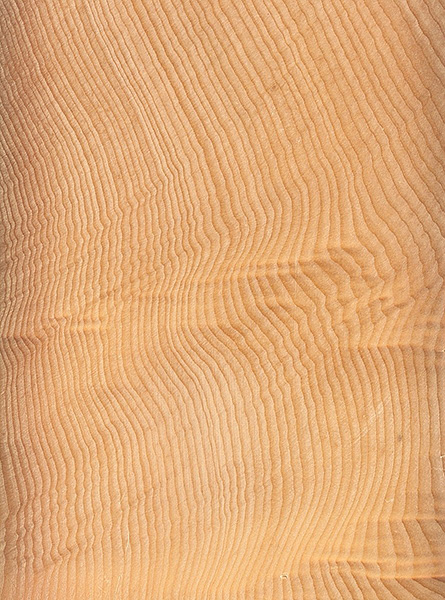The image depicts a close-up view of a piece of wood, likely lumber, featuring an intricate, textured pattern. The surface is primarily orange with reddish-brown hues and is accentuated by vertical lines that are tightly packed and darker than the surrounding wood. These lines follow a wavy, diagonal path, bulging out in the middle before continuing their sinuous journey towards the bottom right. This vertical rectangle image evokes the look of meticulously sanded and carved wood, similar to the ridges formed by tree growth rings, and vaguely reminiscent of a plowed field or undulating sand dunes. The lines, starting from the left and winding down to the right, create a rich, tactile surface that highlights the natural beauty and craftsmanship of the wood.